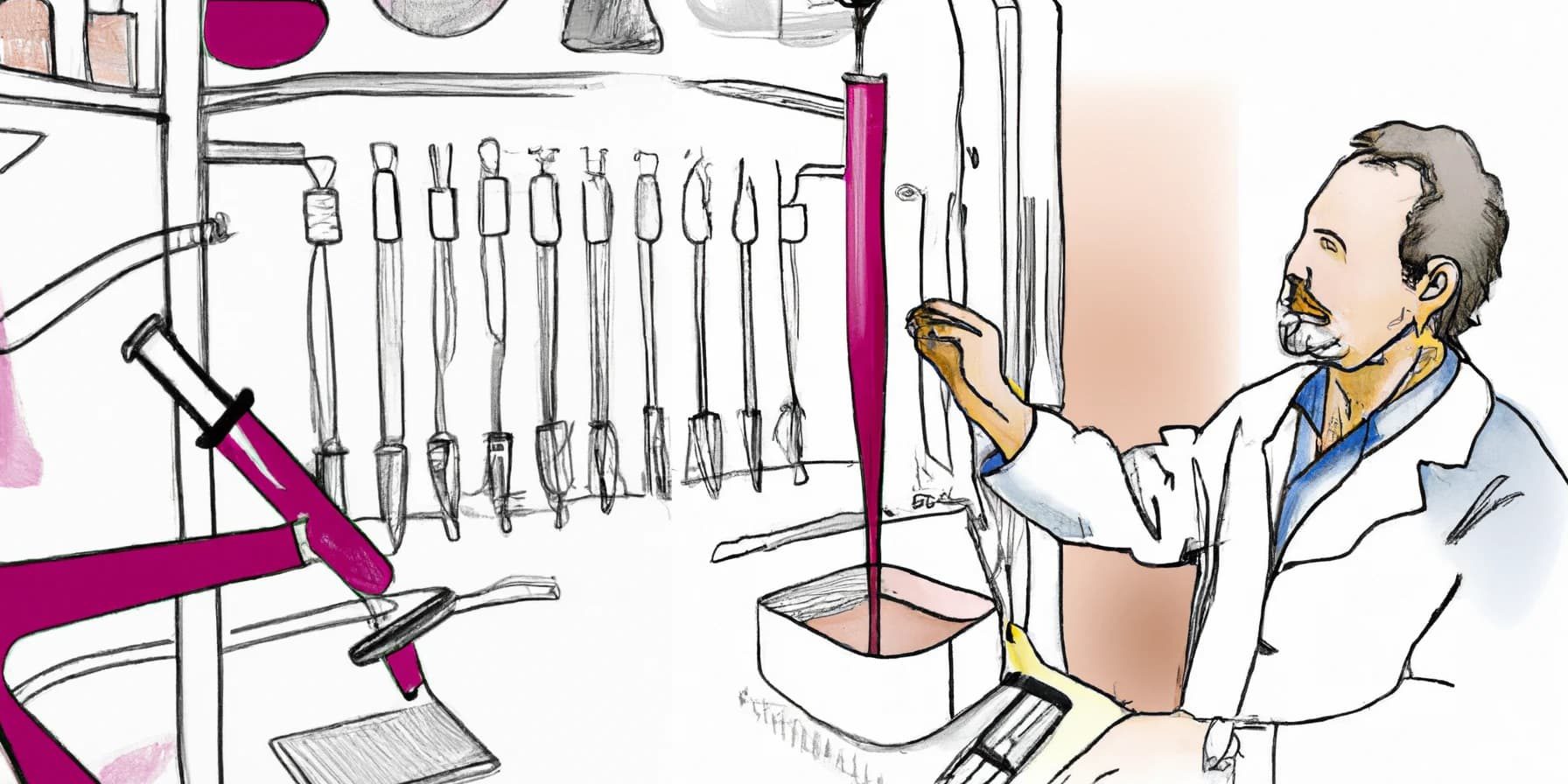In this intricate digital drawing, an older male scientist, possibly in his 60s, is depicted on the right side of a laboratory setting. He is dressed in a white lab coat over a light blue button-down shirt. His brown hair, possibly mixed with gray, peeks out above a somewhat abstract orange or yellowish mustache. His right arm is bent at the elbow, and his right hand is reaching out toward a laboratory setup, presumably grasping for a long, purple-colored tube hanging from the ceiling, which feeds into a container on a table. The scientist's profile reveals a focused expression as he examines his workspace filled with scientific tools. Scattered around him are abstract shapes and apparatuses, including various beakers, large syringes, and a microscope, all predominantly tinted in shades of purple. The backdrop behind him transitions from a darker pink shade to white, emphasizing the laboratory equipment and giving depth to the scene. The overall color palette features white, dark pink, purple, and abstract yellow shadows, lending a surreal quality to the artwork.